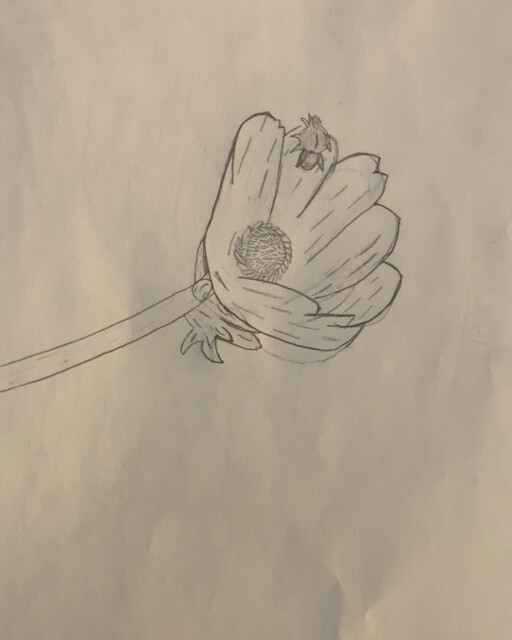This image is a detailed pencil drawing on a plain white piece of paper, possibly appearing yellowish-brown due to the lighting. It features a flower with detailed petals that have lines to indicate depth and folds, centered prominently on the page. From the middle, a long stem extends towards the left, adorned with some leaves at the bottom. The flower's center is filled with numerous tiny strokes, giving it a textured, fuzzy appearance. A small bug, likely a spider or bee, is depicted crawling on one of the petals, seemingly moving towards the center of the flower. Despite its crude and simple style, reminiscent of a child's drawing, the image manages to convey a significant amount of detail and texture.